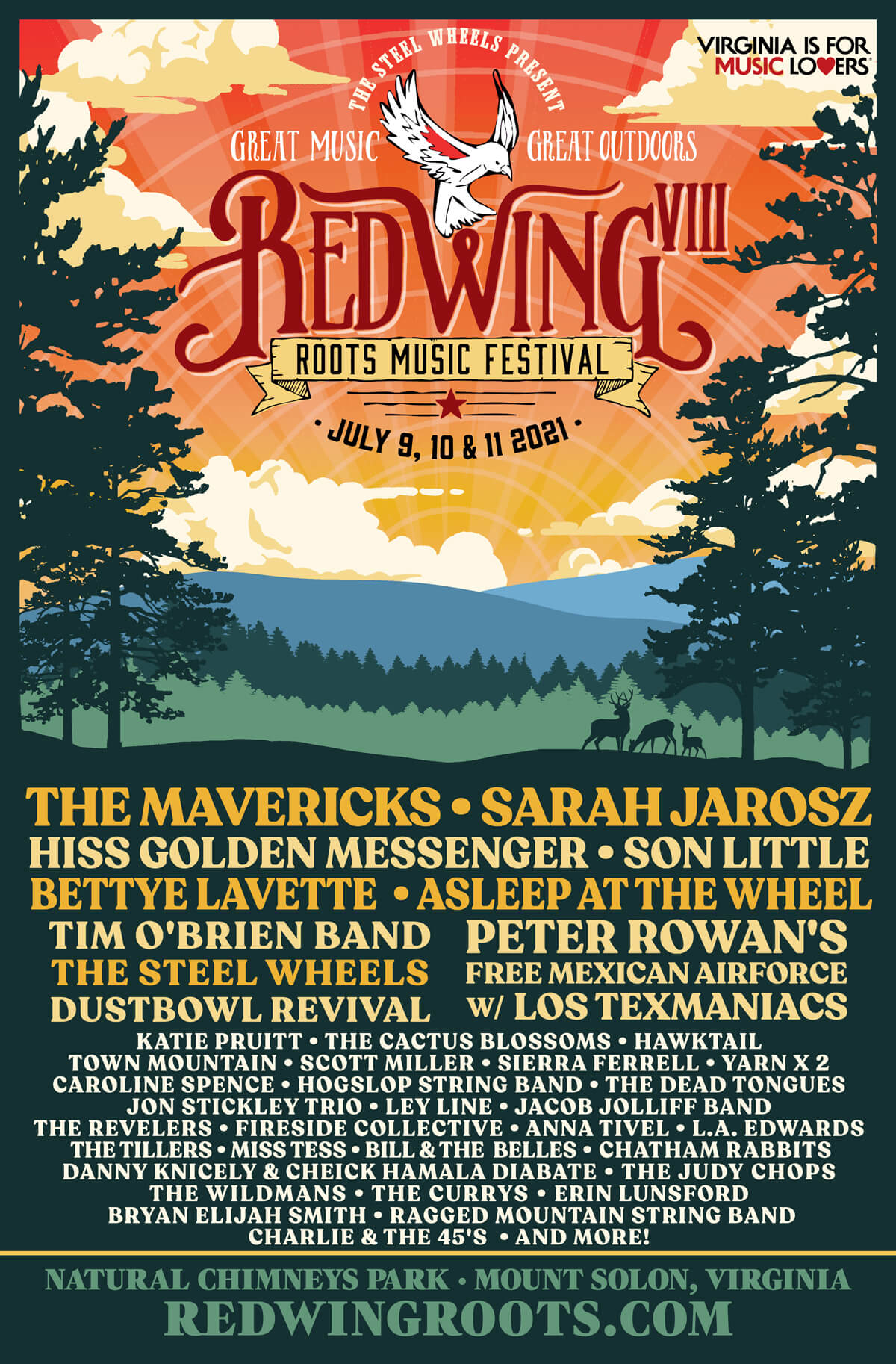The poster for the Red Wing VIII Roots Music Festival, set against a beautiful outdoor forest backdrop with blue mountains and a large, radiant sunset, invites viewers with the motto "Great Music, Great Outdoors." Scheduled for July 9th, 10th, and 11th, 2021, the festival is located at Natural Chimneys Park, Mt. Solon, Virginia. The poster features the event title in red cursive text, accompanied by a white bird graphic over the "W" of "Red Wing." The top of the poster highlights smaller white text stating, "The Steel Wheels Present," while a note in the top right corner adds, "Virginia is for Music Lovers." The artistry is completed by silhouettes of rocks, deer, and trees.

Below the illustration is a comprehensive list of performers, with headliners The Mavericks and Sara Jarosz prominently featured, followed by His Golden Messenger, Son Little, and many more artists in progressively smaller fonts to accommodate the extensive lineup. The bottom section of the poster includes the festival's website, redwingroots.com, for further information.